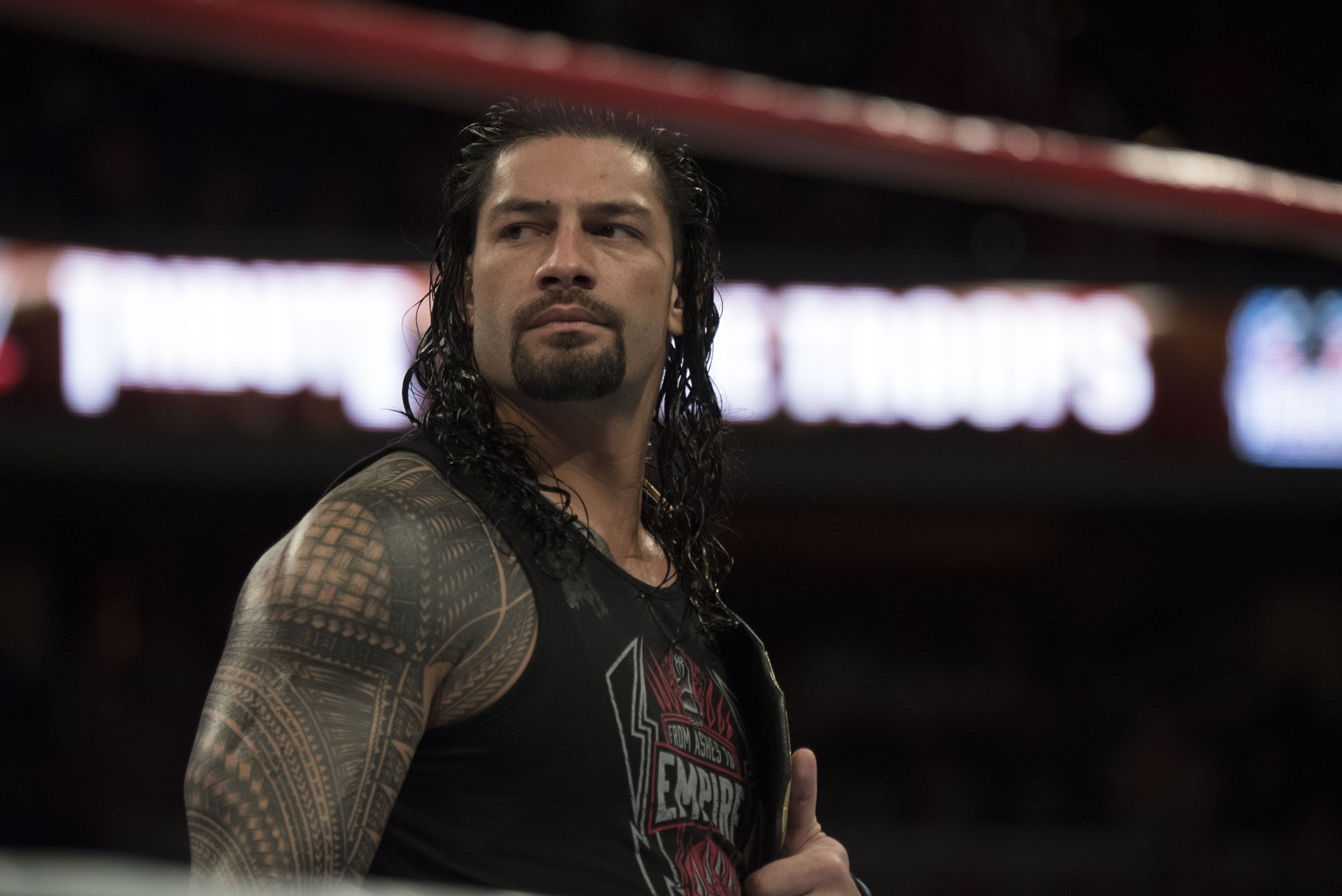This horizontally aligned rectangular photograph captures the renowned wrestler, Roman Reigns. Positioned just left of the center, Reigns, a large man with a muscular build, is seen from the chest up. His long, wet-looking curly black hair drapes over his shoulders, and he sports a black goatee. His serious expression is highlighted by his dark brown eyes, which are directed forward but turned to his left, giving him a contemplative look.

Reigns is wearing a black tank top with a striking red and white emblem that features a lightning bolt design and the word "Empire" prominently displayed. His right arm, adorned with intricate, full-sleeve black tattoos, is clearly visible from the shoulder to just above the elbow. He is giving a thumbs up with his left hand, holding it close to his body.

The background of the image is blurry and somewhat indeterminate; neon lights illuminate the scene, with white lit-up words and possibly a red roof-like structure visible. The upper right-hand corner of the picture is pitch black, adding to the overall dramatic effect of the photo. Additionally, a series of windows can be faintly observed to the left and right of Reigns' head, adding depth to the composition while maintaining focus on the central figure.